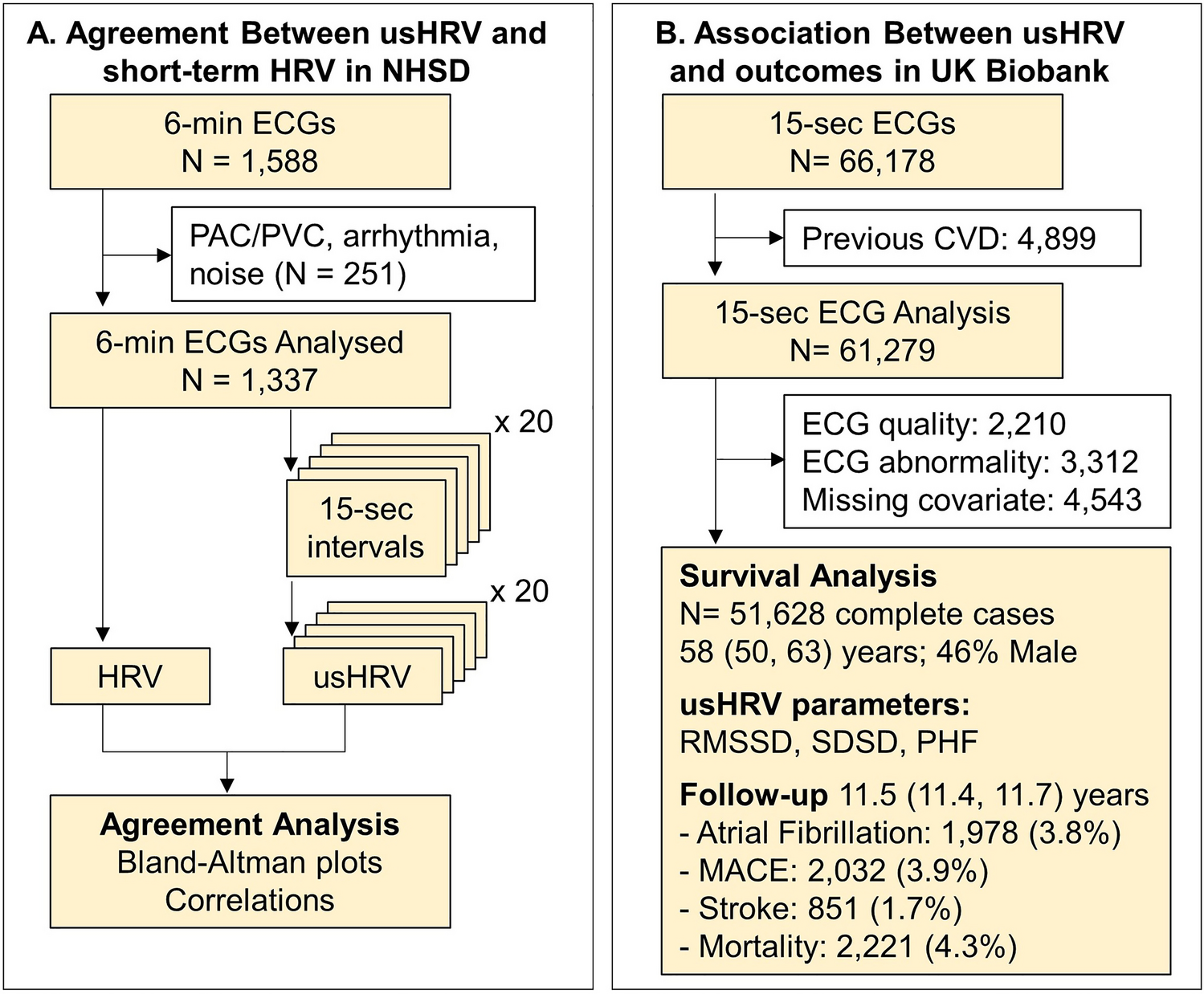The image depicts two detailed flowcharts side by side, each outlined in black and set against a white background. 

**The left flowchart (A)** is titled "Agreement between USHRV and Short-Term HRV and NHSD." At the top, a large white rectangle with black text summarizes this agreement. Beneath it, a beige rectangle notes "6 minute ECGs, N=1,588." Two arrows descend from this point: one directs to a beige rectangle "6 minute ECGs analyzed, N=1,337," and another to a white rectangle stating "PAC/PVC, Arrhythmia, Noise (N=251)." Below the "6 minute ECGs analyzed" rectangle is another beige rectangle labeled "15 second intervals," featuring multiple rectangles behind it, denoted as "Ax20" in black. Another arrow extends left from the "6 minute ECGs analyzed" to a beige "HRV" rectangle, and from the "15 second intervals" rectangle to a "US HRV" rectangle. Both lead to a final white rectangle labeled "Agreement analysis: Bland-Altman plots, correlations."

**The right flowchart (B)** is titled "Association between USHRV and Outcomes in UK Biobank," also starting with a large white rectangle with black text. Below this, a beige rectangle states "15-second ECGs, N=66,178." Similar to the left flowchart, an arrow points downward to "15-second ECG and analysis, N=61,279," with an intermediate white rectangle for "Previous CVD, N=4,899." Below "15-second ECG and analysis," several sub-categories are listed: "ECG quality, N=2,210," "ECG abnormality, N=3,312," and "Missing Covariate, N=4,543." Another arrow points to a larger beige rectangle labeled "Survival Analysis: N=51,628 Complete Cases; 58,506.3 Years; 46% Male." Detailed parameters and follow-up data are listed, including RMSSD, SDSD, PHF, and follow-up periods with specifics on atrial fibrillation, MACE, stroke, and mortality rates.

Both flowcharts use alternating beige and white backgrounds to denote different stages of the analysis, presenting a comprehensive workflow of data assessment, agreement, survival analysis, and outcome correlations in USHRV studies.